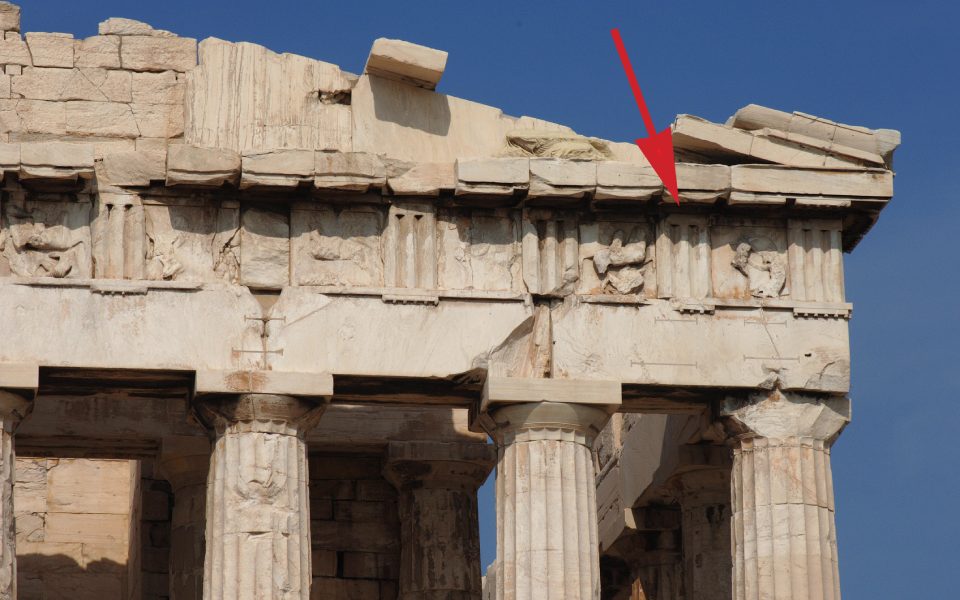The image depicts a fragment of an ancient Greek or Roman building, likely dating back thousands of years. Constructed from stone, the scene includes a partially preserved structure with three prominent stone pillars supporting the roof, and an additional set of three pillars aligned along the inner wall. The building extends from the top left and bottom left corners, slanting downward to the right. The roof appears to be made of stone tiles or bricks, showcasing the enduring architecture of the period. The color palette features various hues, including red, blue, a grayish-white, and a light clay-like reddish tone. In the background, a clear blue sky occupies the right side and top portion of the image, providing a striking contrast to the ancient stone structure in the foreground.